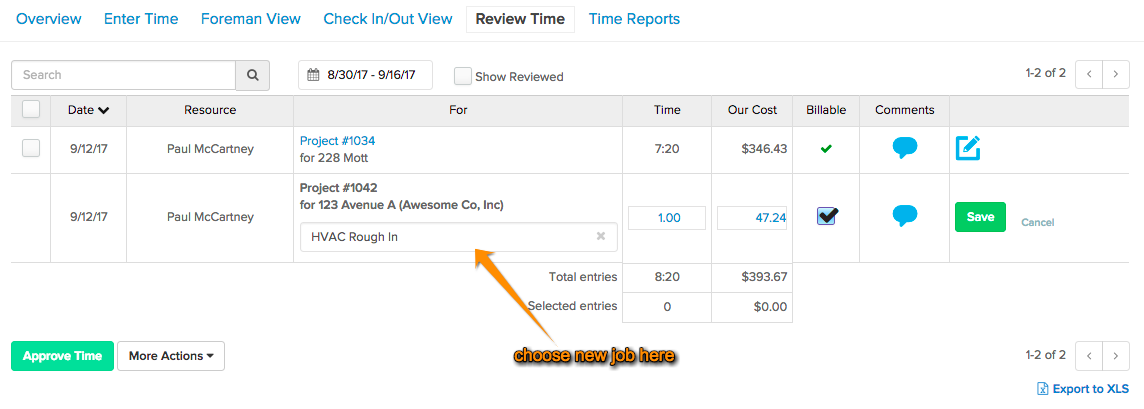The image displays a detailed overview of a time tracking system interface, highlighting various functionalities such as "Enter Time," "Format View," "Check-In," "Check-Out," and "Review Time." The interface currently shows "Page 1 of 2," with entries listed in two rows.

In the first row, the entry details Paul McCartney working on project number 1034 at 228 Mott Street. The second row lists Paul McCartney again, this time assigned to project number 1042 at 123 Avenue A for Awesome Co. Incorporated.

An arrow directs attention to a field in the second row labeled "HVAC Roofing," accompanied by the note: "Choose a new job here." The total cost associated with these entries is $393.67.